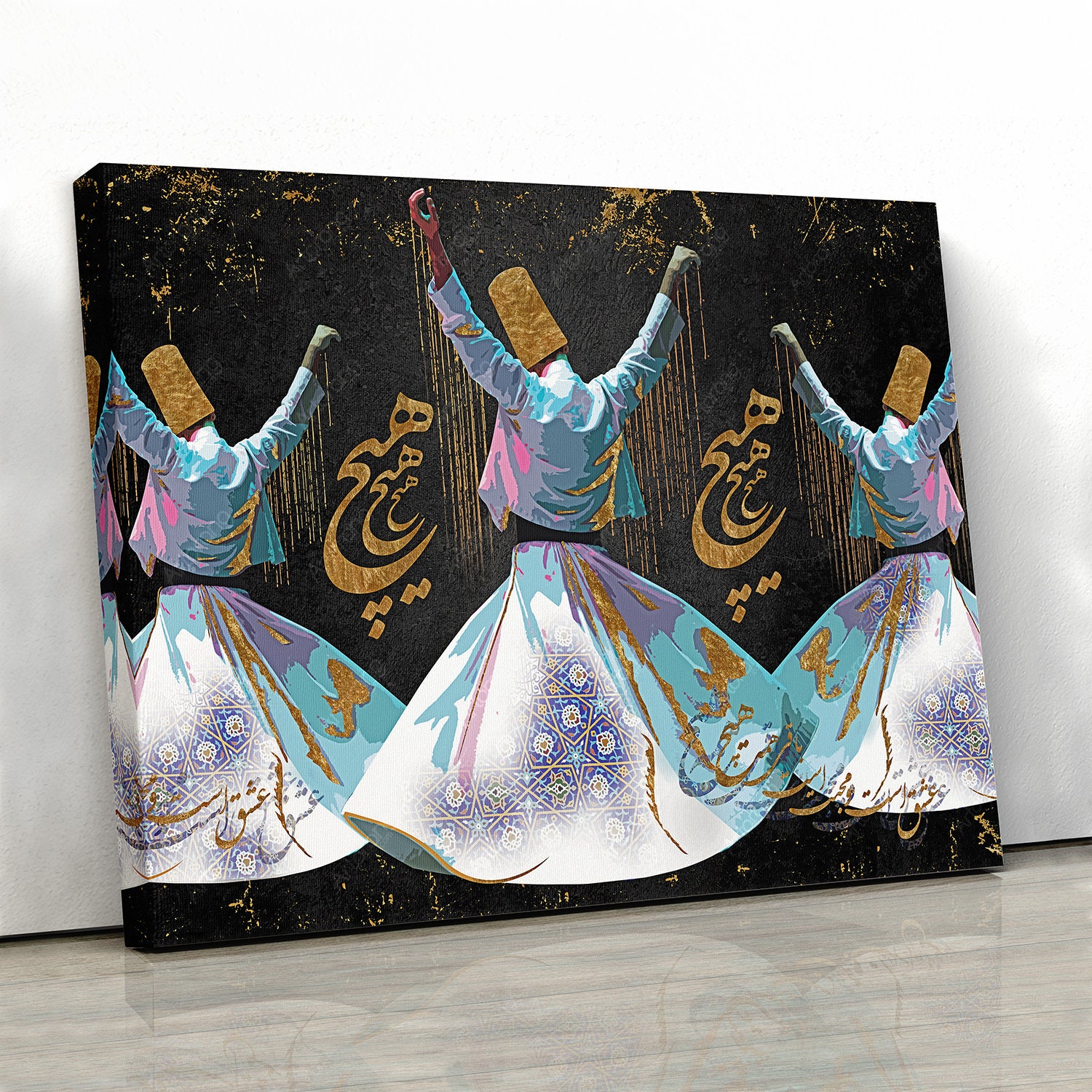The image depicts a rectangular canvas adorned with vivid, artistic illustrations leaning against a pristine white wall on a highly reflective, shiny gray floor. The central focus of the artwork features three panels portraying Sufi dervishes in mid-dance. The dancers are dressed in white garments, consisting of a white shirt and a billowing skirt-like cloth, detailed with gold trim and intricate purple and blue designs. Each dancer wears a tall, cylindrical hat, characteristic of Sufi attire. Their backs are turned, highlighting the flowing, twirling motion of their dance. The canvas itself has a stark black background, embellished with golden Arabic text and sporadically arranged golden spots, adding to the overall ethereal aesthetic.